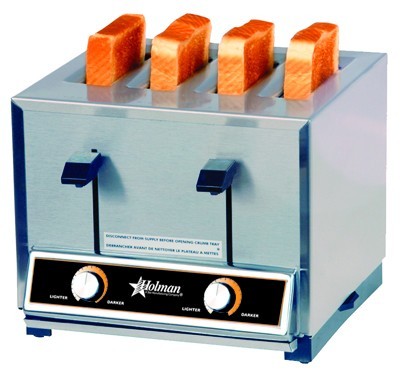This detailed caption combines and refines the various descriptions given into a single, comprehensive summary:

The image portrays a color photograph of a vintage-style toaster set against a stark white background. The toaster, branded "Holman," features a rectangular, industrial design with four slots, each occupied by a thick slice of perfectly toasted, brown bread. The toaster is primarily a bluish-silver hue, although lighting may cast a slight variance in its color. The front panel is black with white trim, and prominently displays the brand name "Holman" alongside a star emblem. Two darker blue handles situated on each side are used to push the bread down into the toaster, while beneath them, two dials allow users to adjust the toast's doneness from lighter to darker. These knobs have a white circle on the left and a red circle on the right, indicating heat levels. The overall appearance of the toaster evokes a nostalgic, mid-20th-century aesthetic, reminiscent of imagery from fifties or sixties magazines. The thick slices of toast, possibly Texas toast, exhibit an unnatural orangish shade, ensuring they stand out in the otherwise minimalist composition.